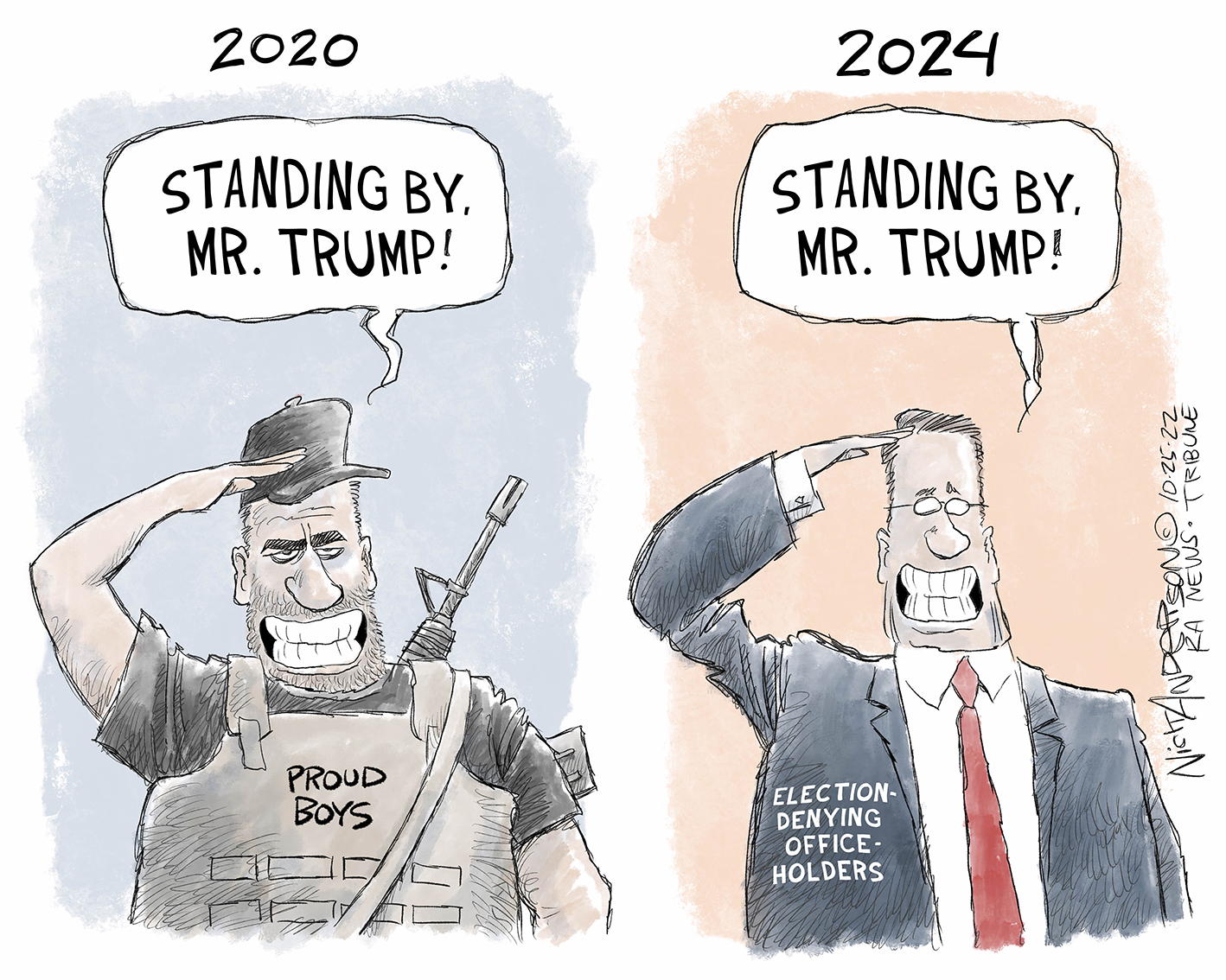This political cartoon is divided into two panels, each representing different years. The left panel, labeled "2020," features a man in military-style body armor emblazoned with the text "Proud Boys." He is shown saluting with his hand above his hat but not quite to his eyebrow, his arm clutching an automatic rifle slung over his shoulder. He has a stubbly beard and a wide, toothy smile, with thick eyebrows adding to his rugged appearance. A speech bubble above him reads, "Standing by Mr. Trump."

The right panel, shaded in an orangey-salmon color and labeled "2024," depicts a different man mimicking the same salute. This man is dressed in a black suit, a red tie, and wears glasses. His suit jacket bears the text "Election Denying Officeholders." He too has an open-toothed grin, and a speech bubble echoes the previous one, stating, "Standing by Mr. Trump."

The cartoon juxtaposes the two figures to highlight the transformation and continuity in support for Mr. Trump over the years, from a rugged militant supporter in 2020 to a polished political figure in 2024.